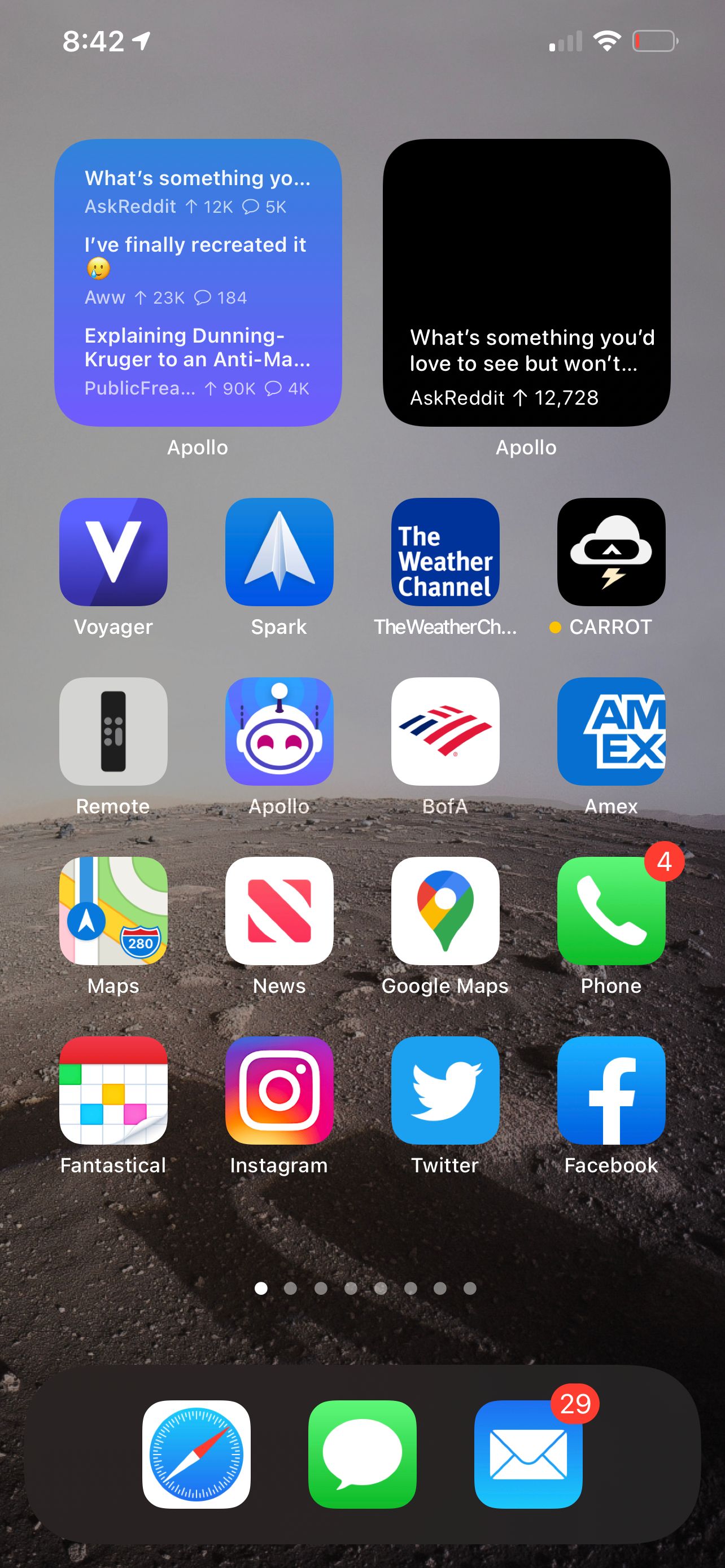The image showcases an iPhone displaying a website, with several key details visible. The battery indicator at the top right corner shows a critically low charge, highlighted in red, and the Wi-Fi connection is weak, indicated by a single bar. The time displayed on the phone is 8:42. 

On the screen, there's a blue text box on the left side with the partially visible text, "What's something you?" The current webpage is an Ask Reddit thread with the header, "What's something you'd love to see but won't?" in black text. The subreddit and user information underneath is tagged with "Apollo."

The rest of the screen displays an assortment of app icons in two sections. The upper section includes apps such as Voyager, Spark, The Weather Channel, Carrot, Remote, Apollo, BotA, Amex, Maps, News, Google Maps, Phone, Fantastical, Instagram, Twitter, and Facebook. At the bottom of the screen, docked apps include Safari, Messages, and an email app, which has a notification badge displaying the number 29 in a small red circle.